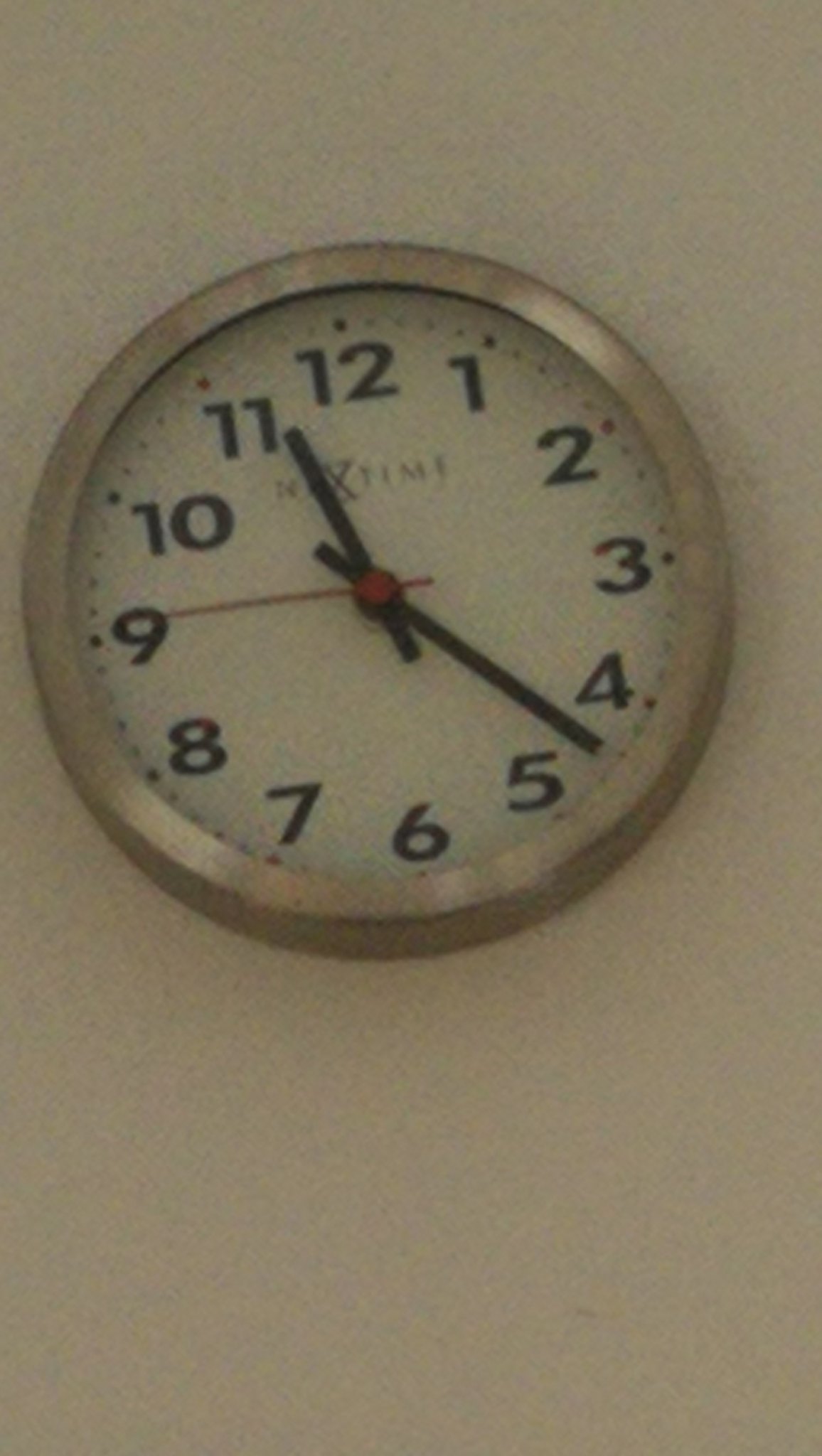This photograph showcases a round analog clock mounted on a light-colored wall. The clock features a frame crafted from brushed stainless steel, giving it a sleek, modern appearance. The clock face displays the time as 11:22, with black numbers from 1 to 12 arranged in a classic circular format. Small black dots mark each second. The hour and minute hands are thin, elongated black rectangles, while the second hand is a slender, needle-shaped red pointer, adding a subtle yet vibrant contrast to the overall design. The image captures the elegance and simplicity of the clock's aesthetic against the neutral backdrop of the wall.